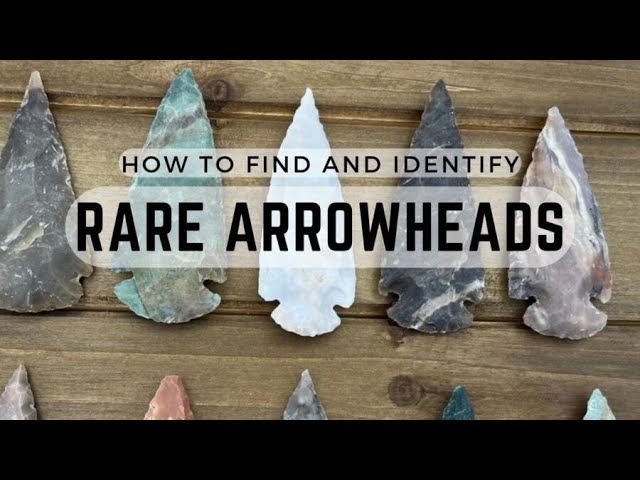The image features a centered photograph bordered by solid black banners across the top and bottom. The photo itself is about five inches wide and three inches high, showcasing a worn, horizontal slatted wooden surface in a light brown color with varying shades due to the wood grain. On this surface, there are two horizontal rows of arrowheads, each row containing five arrowheads aligned side-by-side. 

In the top row, from left to right, the arrowheads are: a grayish one with a hint of white, an aqua-colored one, a completely white one, a marbled one with larger streaks of dark gray and white, and one that is a blend of lighter colors. The bottom row displays only the pointed tips of the arrowheads. Overlapping the image, two transparent gray horizontal ovals contain black text that reads, "How to find and identify" on the top oval, and "rare arrowheads" in larger font on the bottom oval. The arrowheads themselves are various in size and shape, resembling Christmas trees.